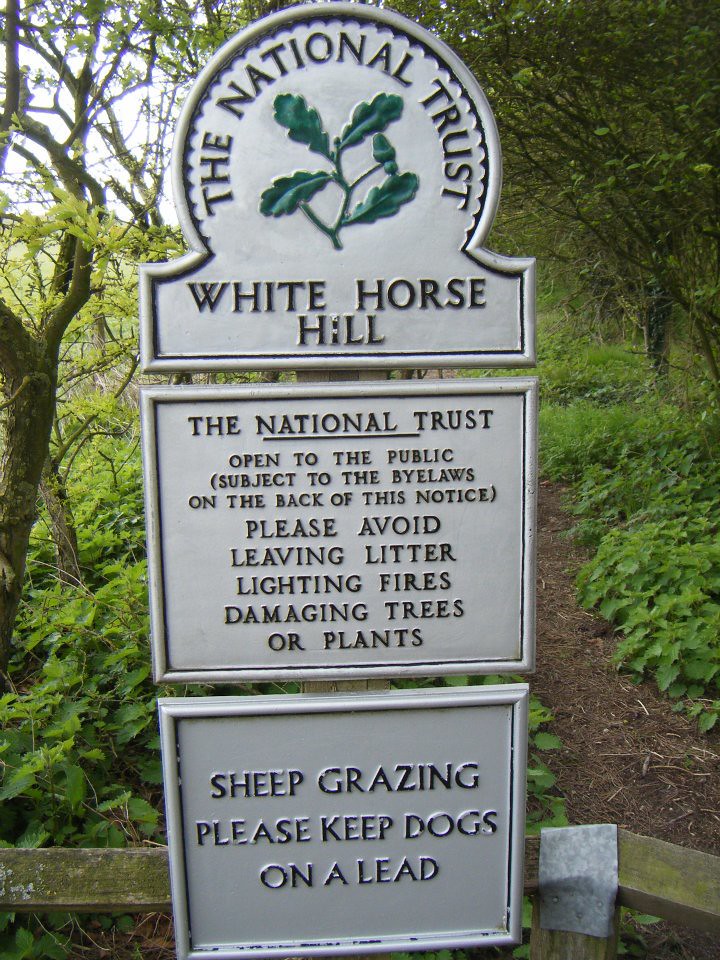This photograph captures a three-part sign in a public park, prominently situated in front of a wooden fence. The top section of the white, silver sign is rounded and displays the National Trust logo in green text alongside an illustration of a branch with leaves. Below the logo, it reads "White Horse Hill." The middle section is square and states, "The National Trust. Open to the public subject to the bylaws on the back of this notice. Please avoid leaving litter, lighting fires, damaging trees or plants," also in green text. The bottom square part of the sign advises, "Sheep Grazing, please keep dogs on a lead." The sign is mounted on a post, flanked by greenery which includes low shrubs at the base, and branches and leaves extending upwards. There is also a dirt path visible leading further into the park.